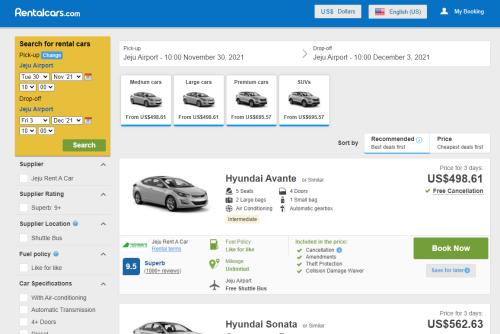The image consists of a detailed web interface for booking rental cars. 

**Header Section:**
- A blue rectangle spans the top of the image. On the left, it displays the logo "rentalcars.com." To the right, there are two white sections. The first contains some text, and the second features an American flag and additional words.

**User Interaction Section:**
- Below the header, a gray rectangle houses multiple interactive elements.
  - On the left, an orange rectangle contains text — some black, some red.
  - Adjacent to it, a smaller blue rectangle displays a single word.
  - Several white rectangles appear throughout, suggesting spaces for inputting dates.
  - Text elements are interspersed in black and green fonts.
  - Another defined area at the bottom features a green rectangle labeled "Search."
  - To the right of it, a long white rectangle also contains dates, separated by an arrow.
  
**Car Listings Section:**
- Four white squares, each showing a picture of a car and labeled with blue text, appear underneath the interaction section.
  
**Informational Sidebar:**
- On the right, white rectangles with text, highlighted by blue lines at the bottom.
  
**Options Section:**
- On the left side, a sequence of white squares with words next to arrows pointing up.
  
**First Car Listing:**
- A white rectangle shows an image of a car labeled "Hyundai Avante."
  - Symbols are placed below, in two rows of three, with descriptive text.
  - On the right, it mentions "US$498.61" followed by a check mark and additional words.
  - Under the symbols, a small yellow rectangle with some text, followed by a green symbol with a green word.
  
**Additional Information:**
- Below, a blue square containing numbers is paired with blue and black text.
  - There is also a green-outlined rectangle partially filled with green, alongside green words.
  - This section includes symbols for maps and airplanes with respective text.
  - A list with green check marks and black text appears, the top checked item marked with a blue dot.
  
**Call to Action:**
- On the right, a green rectangle prompts to "Book Now," followed by a gray rectangle with text in blue.
  
**Second Car Listing:**
- Just visible at the bottom is another white rectangle showing part of a car image labeled "Hyundai Sonata," with words on the right and "US$562.63" underneath.

This caption elaborately describes the layout and content of the web interface for booking rental cars, detailing each interactive and informational element presented.